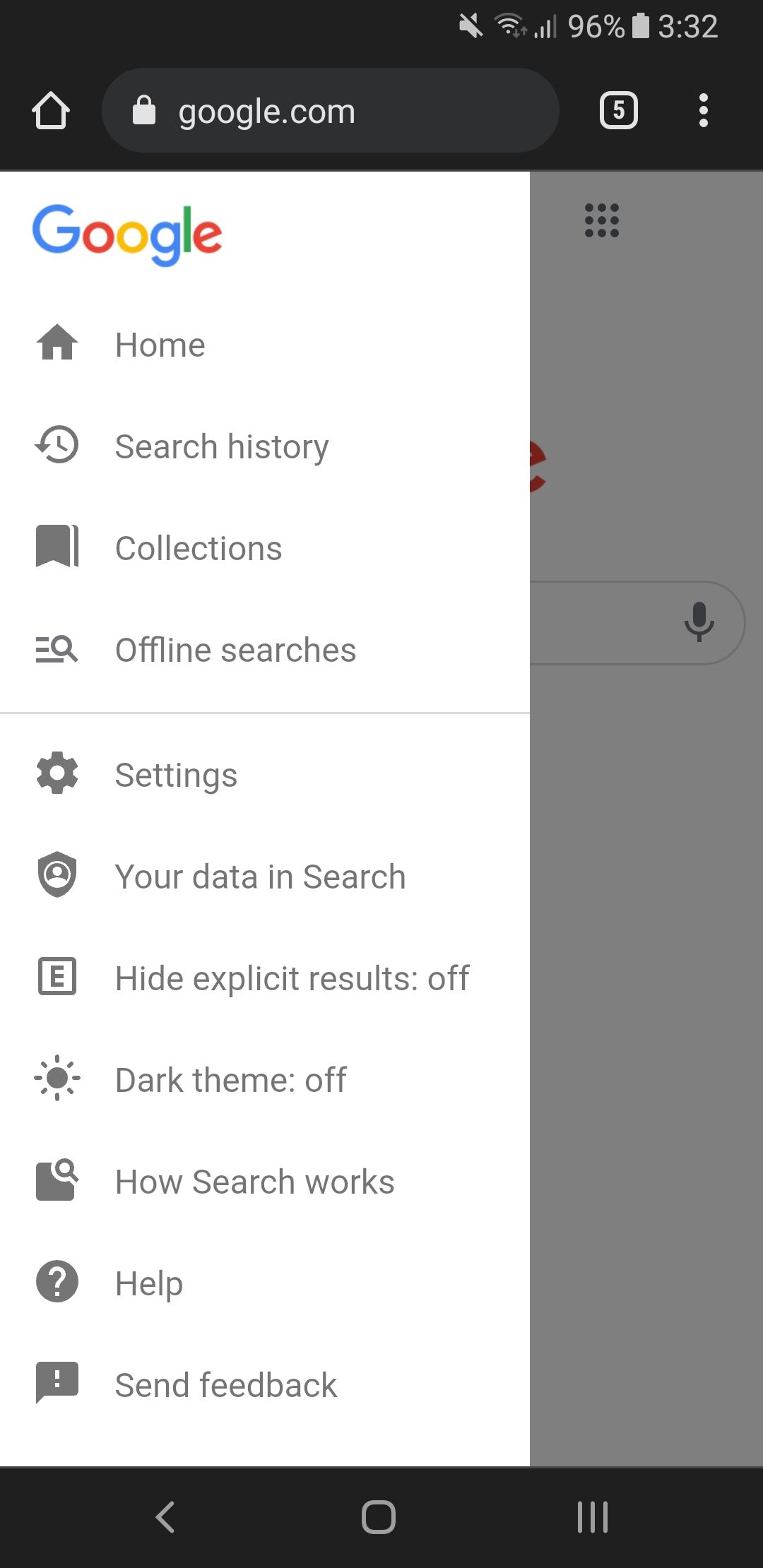This image is a detailed screenshot of the sidebar menu in the Google search application. 

On the left, the sidebar displays a list of menu options: 

- **Home** with a house icon.
- **Search History** marked by a clock icon rewinding time.
- **Collections** featuring two folder icons.
- **Offline Searches** represented by an hourglass or magnifying glass icon.
- **Settings** indicated by a gear icon.
- **Your Data in Search** symbolized by a shield with a human silhouette.
- **Hide Explicit Results** with an "E" inside a square (currently set to off).
- **Dark Theme** shown by a sun icon (currently off).
- **How Search Works** depicted with a magnifying glass over a dark square.
- **Help** marked by a white question mark inside a gray circle.
- **Send Feedback** shown with an exclamation mark in a gray speech bubble.

The URL bar at the top displays "google.com" with a small lock icon, indicating the website is secure. The status bar at the top of the phone screen shows a battery level of 96%, the time as 3:32, and connectivity indicators: a Wi-Fi icon and three out of four network bars. The familiar Google logo is also visible at the top of the menu.

Each menu option is accompanied by its respective icon for easy identification, providing users with access to various features and settings within the Google search application.